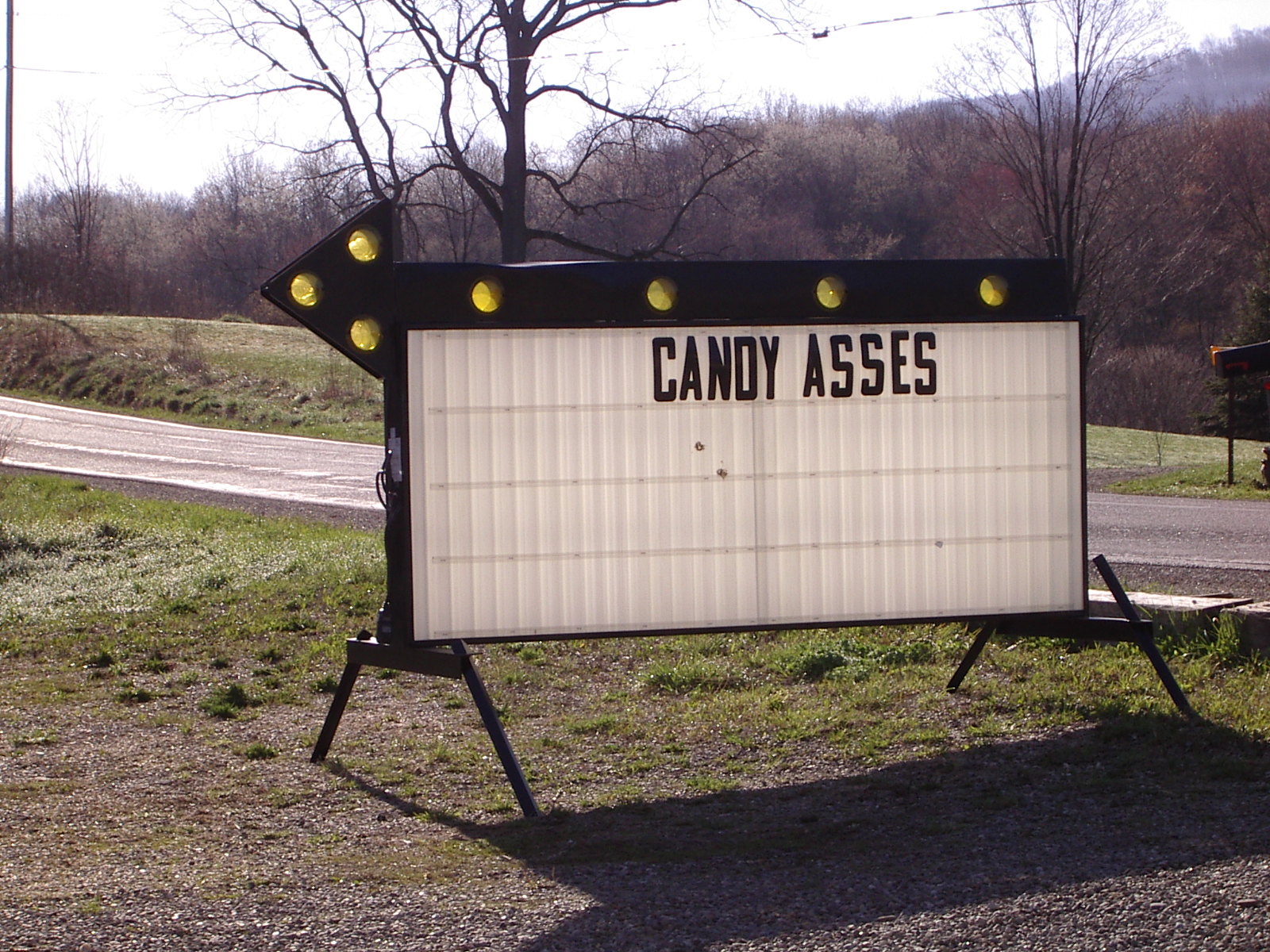The image captures a detailed roadside scene featuring an illuminated sign. The sign, supported by a sturdy metal frame with four legs, stands prominently on a gravel patch beside a country road. It has a black strip at the top with an arrow pointing left, outlined by four yellow lights along its shaft and three additional lights at the arrowhead. The main body of the sign is backlit white and displays the phrase "Candy Asses" in bold lettering. The background reveals a contrast in seasonal foliage: leafless trees directly behind the sign, while a dense stand of trees adorned in vibrant fall colors—predominantly orange—extends to the right and across the scene. Additionally, a larger hill rises in the distance to the right, adding depth to the rural landscape.